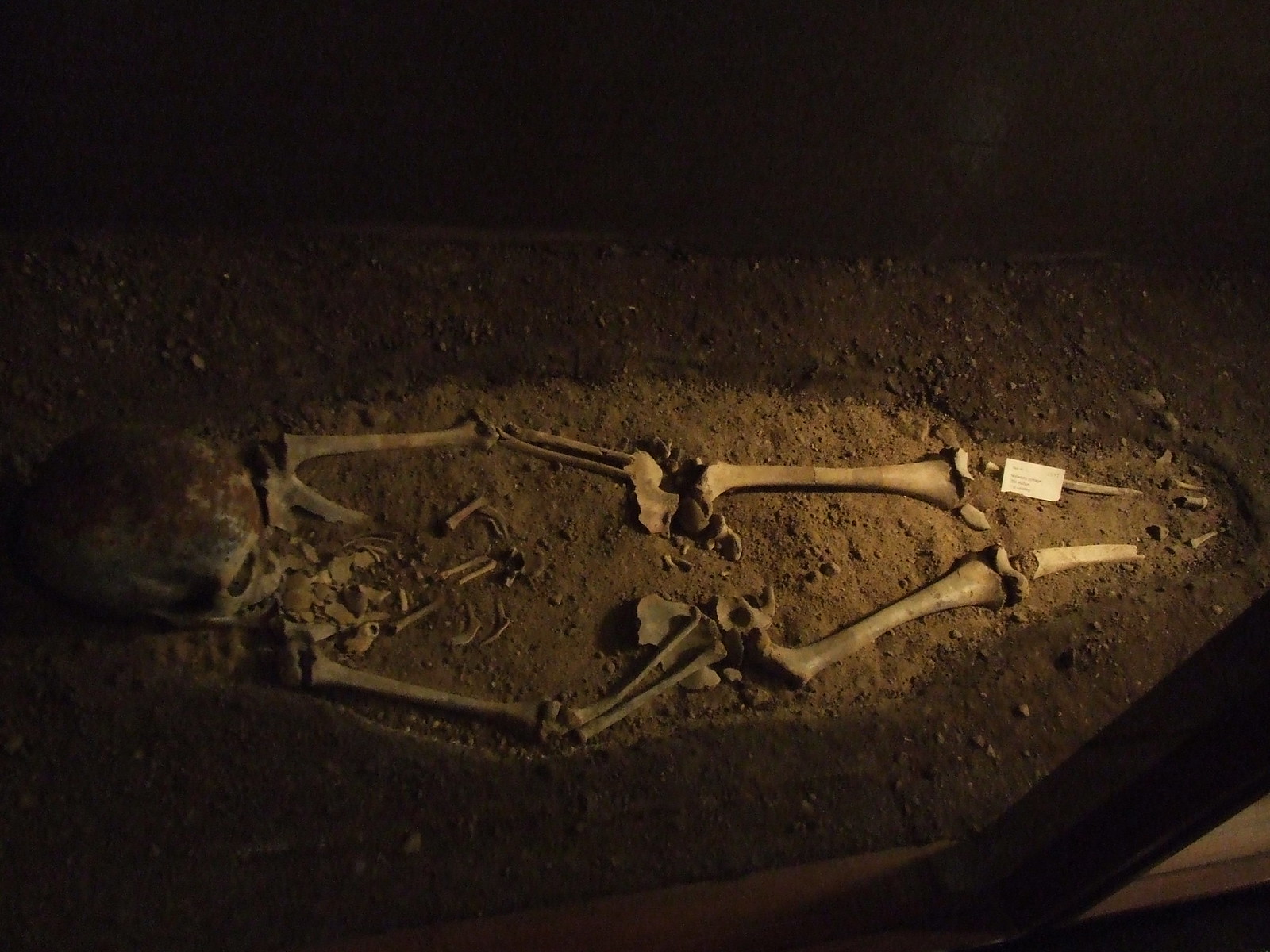The image is a detailed photograph likely taken in an indoor archaeological setting or museum. It captures a grave illuminated from above, surrounded by dark, shadowy edges. The photograph, rectangular in shape and oriented horizontally, displays a skeletal remain partially buried in dirt. Starting from the bottom left and extending to the upper right, a brown divider and a pole attempt to segregate and protect the area of interest. At the center lies an oval impression in light brown dirt, encircled by darker soil. Inside this oval, the skeleton is arranged with the skull facing right, and the femurs, arms, and additional leg bones extending below it. The ribcage appears largely incomplete, with only a few small bones remaining, and the pelvis seems either buried or crushed by the surrounding dirt. The feet are not visible. There is also a noticeable small white card with black print near one of the smaller leg bones, but the text is too indistinct to read. The upper portion of the image fades into darkness, emphasizing the illuminated grave site below. The scene may be viewed through a clear case, suggesting a controlled environment such as a museum exhibit.